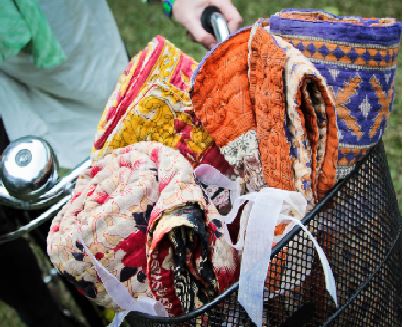This outdoor photograph primarily features a black wire mesh basket mounted on the front handlebars of a bicycle. The basket is filled with four rolled-up, vibrantly colored textiles, which appear to be quilts or embroidered rugs. The bicycle itself has visible handlebars, a small bell, and is ridden by a woman, although only her left hand and part of her white dress are visible. The scene is set against a backdrop of green grass. The textiles in the basket are each distinctive: the one on the left displays a pattern of roses, the one furthest back features yellow and pink hues, the one in the front combines orange and white with black accents, and the one on the upper right showcases an intricate design resembling Indian or Navajo patterns with orange X-shaped crosses shaded in purple.